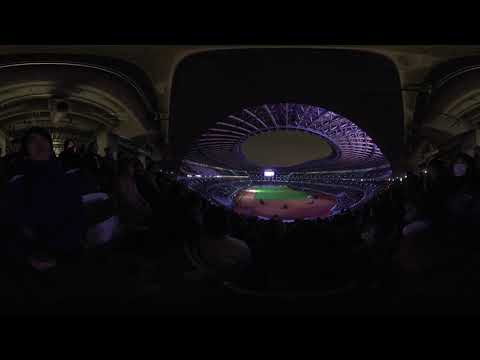The photograph captures a bustling baseball stadium at dusk, taken from the bleachers using a fisheye lens, which distorts the image into a rounded, eyeball-like shape. The viewpoint is notably far from the field, emphasizing the distance and giving an encompassing view of the structure. The roof of the stadium is fully open, and intricate bracing with large steel beams forming X shapes is visible on top. Despite the darkness that envelops the bottom half of the image, the field’s dirt and green sections are discernible in the center, surrounded by expansive bleachers stretching from first to third base. To the left, some circular shapes are faintly visible, their forms warped and unclear due to the lens effect. Bright lights shine down, illuminating the field and creating a stark contrast against the dark surroundings.